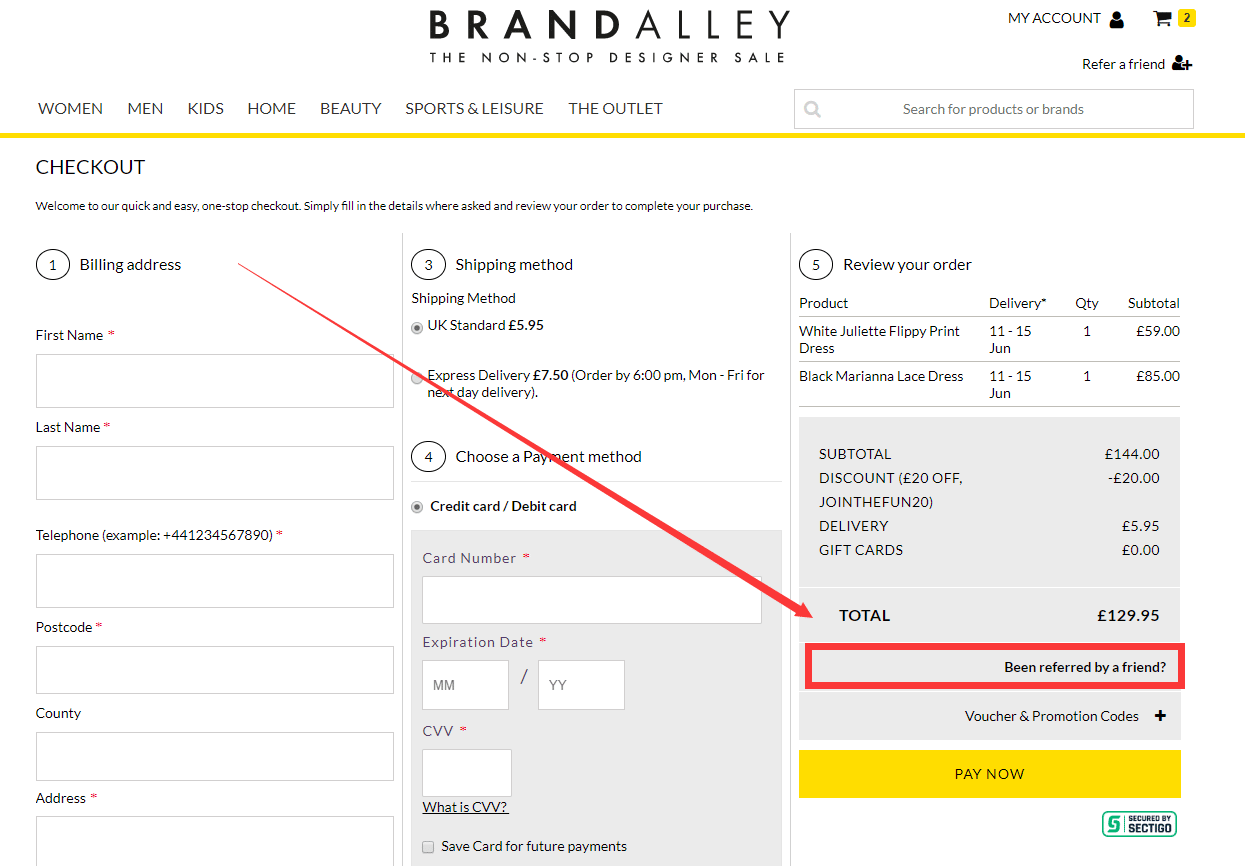This image, sourced from the website Brand Alley, prominently features their tagline "The Nonstop Designer Sale." At the top of the page, a navigation bar provides clickable categories for "Women," "Men," "Kids," "Home," "Beauty," "Sports & Leisure," and "The Outlet." Additional icons include "My Account," a shopping cart indicating two items, a "Refer a Friend" section, and a search bar for products or brands. 

The central focus is on the checkout page, detailed with a step-by-step guide for completing a purchase. It warmly welcomes users to their "quick and easy one-stop checkout." There are fields for entering personal information, including first name, last name, telephone number, postcode, county, and address. 

The checkout process continues with selecting a shipping method, offering options like UK Standard and Express delivery. Next, users can choose a payment method, entering their card information such as card number, expiration date, and CVV. 

Finally, the order review section details the costs involved: items totaling £144, a £20 coupon applied, with an additional delivery charge of £5.95, bringing the total to £129.95. An eye-catching red box with an arrow highlights the "Been referred by a friend?" section.